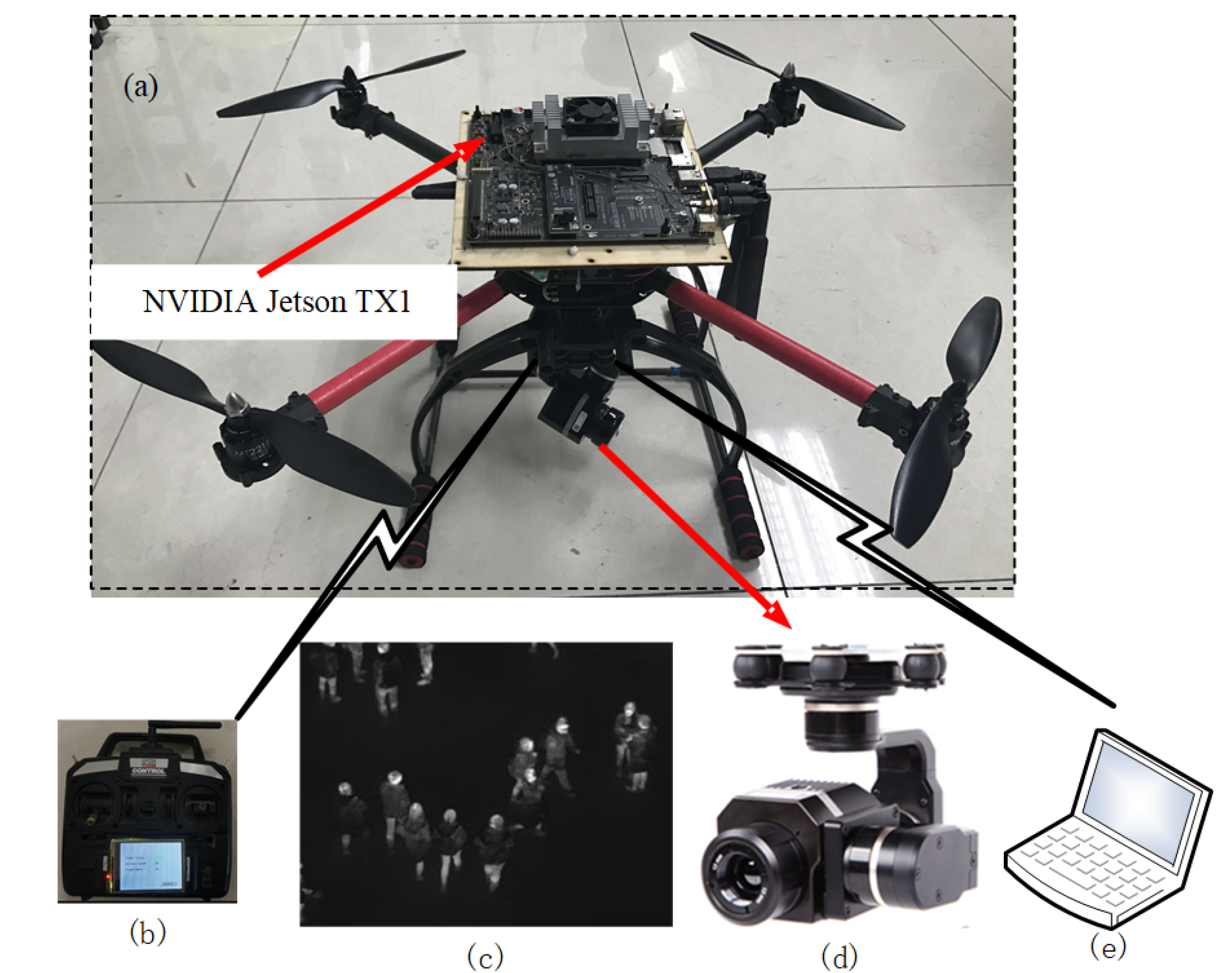This infographic consists of five distinct visual elements labeled A through E. Image A, which is the largest and located at the top, is a color photograph of a substantial drone equipped with a camera, reminiscent of a GoPro. This drone features a black base with two red arms and two black arms, all equipped with propellers. On top of the drone is a circuit board labeled "NVIDIA Jetson TX1," highlighted by a white box with black text and a red arrow pointing to it. This circuit board appears to be a sophisticated computing unit, possibly equivalent to a motherboard, but with specialized ports and no PCI Express slots. The drone itself is positioned on a white tile floor and includes four landing legs attached to a bar, resembling helicopter landing gear. 

Beneath Image A, there are four smaller images arranged in a row from left to right. Image B is a close-up of the drone's remote control, featuring a small LCD or LED screen at the bottom. Image C is a night vision photo showing people walking, with the subjects highlighted in light colors against a dark background. Image D depicts the camera mounted on the drone, showcasing its attachment mechanisms. Lastly, Image E is a simple vector drawing of a laptop, appearing more illustrative and less realistic, possibly resembling a calculator in its simplicity.